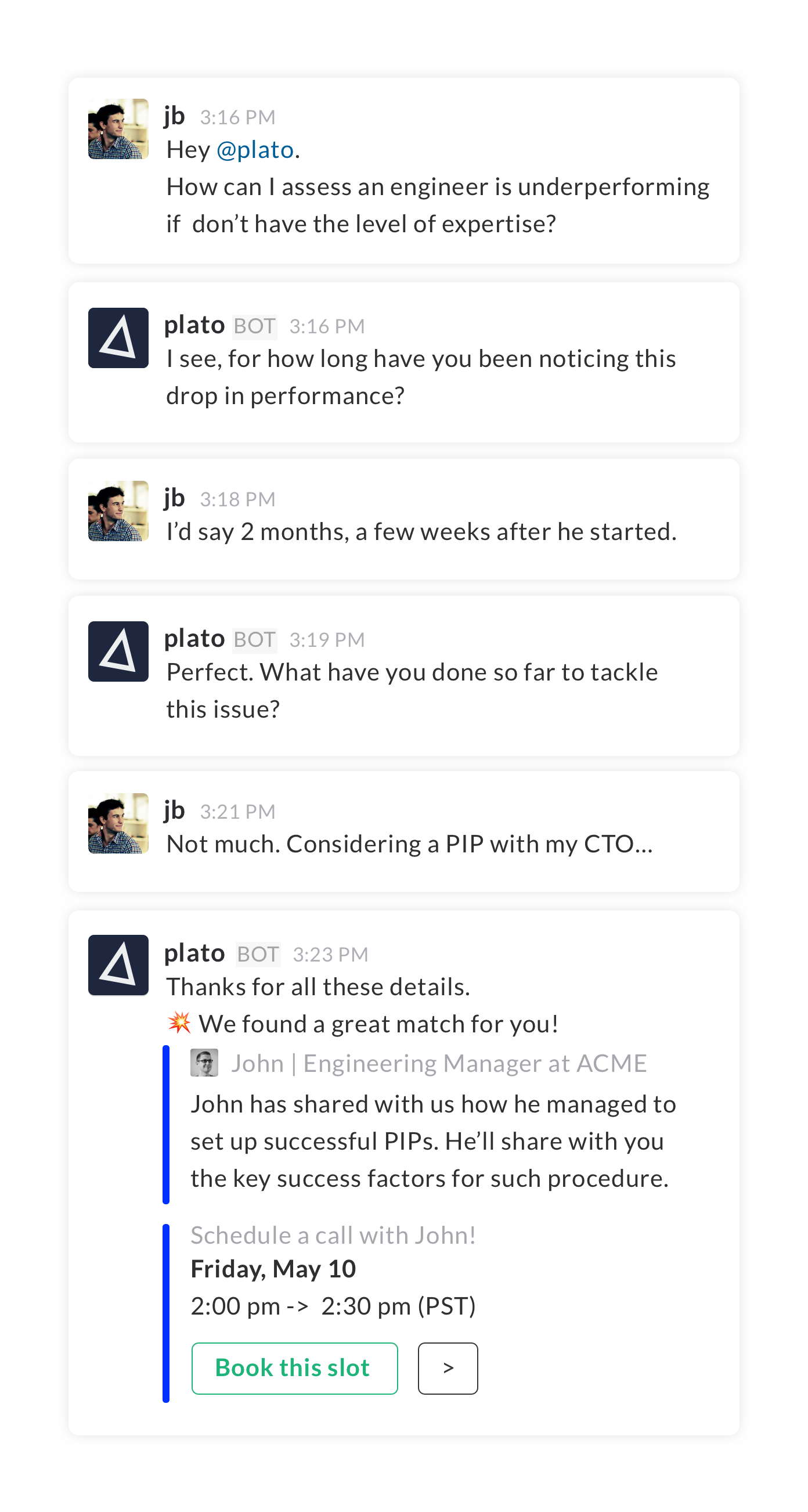The image depicts a white background with a text-based conversation resembling a chat log, likely from a customer service interaction or a vlog page. The conversation is displayed vertically, following a sequential order from top to bottom.

At the start of the chat, the user identified as "JB" initiates the conversation at 3:16 pm, asking: "Hey Plato, how can I assess if an engineer is underperforming if I don't have that level of expertise?" Plato, an automated bot, responds by inquiring, "I see, for how long have you been noticing this drop in performance?" 

JB replies, "I'd say two months, a few weeks after he started." Plato then asks, "Perfect, what have you done so far to tackle this issue?" JB responds, "Not much, considering a PIP with my CTO."

Plato acknowledges the information provided and offers a solution: "Thanks for all these details. We found a great match for you: John, Engineering Manager at Acme. John has shared with us how he managed to set up successful PIPs. He will share with you the six key success factors for such procedures. Schedule a call with John on Friday, the 10th of May, from 2:00 pm to 2:30 pm PST." 

At the bottom of the conversation, there is a green button labeled "Book this slot."